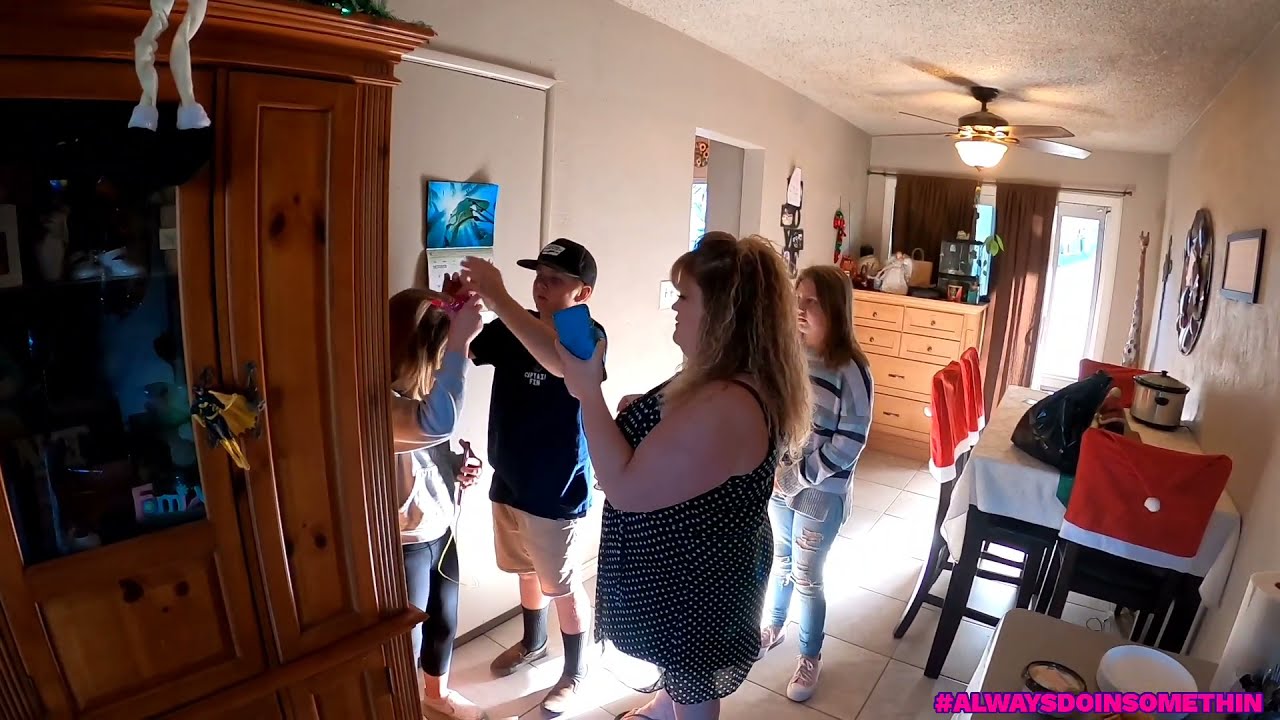The indoor photograph captures a candid moment in a family’s living room during the daytime, illuminated by both natural light through a sliding glass door with round curtains and artificial light from a ceiling fan. Centrally positioned is the mother, a slightly overweight white woman with brown hair dyed blonde and highlighted, dressed in a black sundress with white polka dots, holding a blue cell phone in her left hand. To her right, a young white girl with brown hair, wearing a blue sweater and distressed blue jeans, observes the interaction. On the mother's left, a boy in a black hat, black shirt, and white shorts reaches over the head of another girl. This girl, standing next to a brown wooden hutch with a TV emerging from it and a Batwoman figurine hanging from one of its knobs, has blonde hair and is wearing a white sweater and black leggings. She appears to be fixing something on her head. The room features a standard setup with a ceiling light, white walls, a closet, furniture, and a calendar on the wall. Adding a festive touch, the chairs around a dining table are adorned with Santa hat covers. The bottom right of the image includes the hashtag “#alwaysdoing something” in pink font with a purple border.